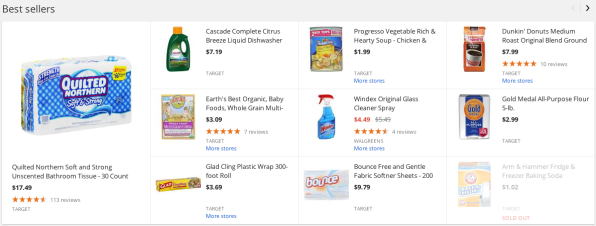The image is a visually organized grid layout displaying various best-selling products under the header "Best Sellers," which is presented on a gray background with black text. The grid is situated within a horizontally long rectangle, and each product resides in its own smaller rectangle against a white background. 

Highlighted sections include:

- **Quilted Icons:** Featuring various household items.
- **Cascade Complete Citrus Breeze Liquid Dishwasher Detergent:** Listed among items available for purchase.

Among the products displayed are:

1. **Windex Original Glass Cleaner Spray**
   - **Visual Description:** A clear plastic bottle containing blue liquid, labeled with the Windex logo on a blue sticker.
   - **Price:** $4.49
   - **Reviews:** 4.5 stars based on four reviews.
   - **Availability:** Can be purchased at Walgreens.

2. **Dunkin' Donuts Medium Roast Original Blend Ground Coffee**
   - **Visual Description:** Standard packaging for ground coffee.
   - **Price:** $7.99
   - **Reviews:** Rated 5 stars based on five or ten reviews.
   - **Availability:** Available at Target.

Most products featured in the grid can be purchased at Target, providing shoppers with location options. The overall design is user-friendly, emphasizing the products through a clean and structured presentation.